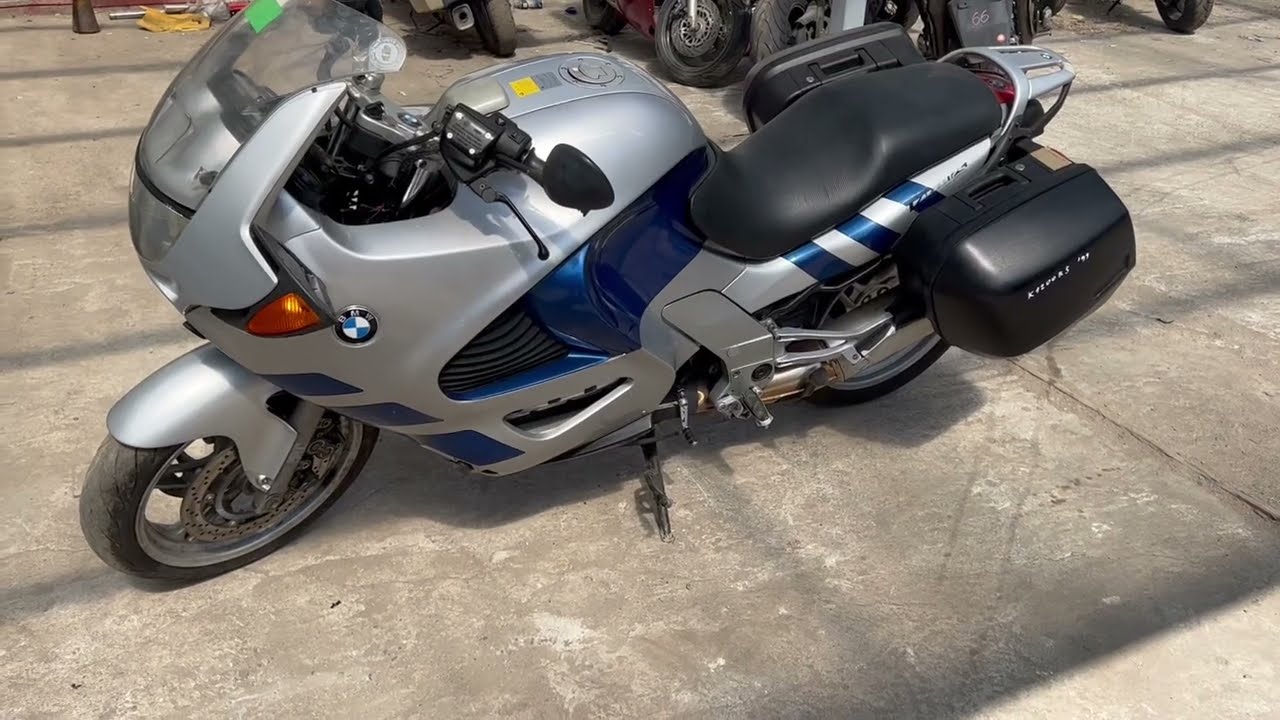This photograph features a modern BMW touring motorcycle, prominently positioned in the center of the image on a stone or asphalt roadway. The motorcycle, primarily silver with black accents and blue highlights, includes a black seat and two black storage compartments flanking the sides behind the back seat. The front end of the bike is equipped with a wind guard and additional coverings that might conceal the engine, along with a small BMW emblem. The scene appears to be outdoors during the day, possibly at a bike dealership or mechanic lot. In the background, there are the front tires of other motorcycles, indicating a parking area, with no people present in the photograph.